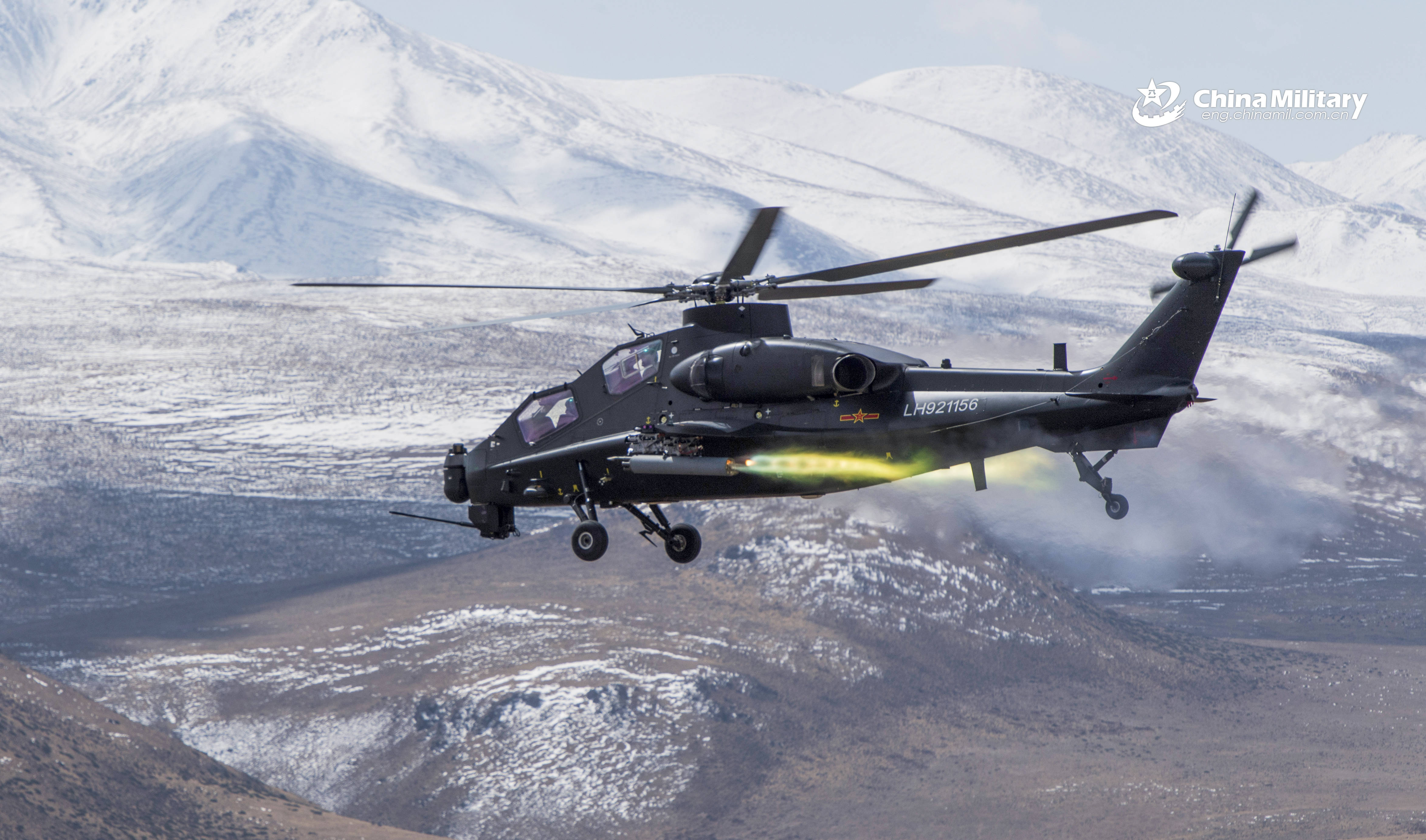This image showcases a dark gray Chinese military helicopter emblazoned with a Chinese flag and the text "China military" in the upper right corner. The helicopter, mid-flight with its landing gear deployed, features a large primary rotor on top and a smaller tail rotor. Details include white lettering, presumably its model number, and a distinctive yellow marking on the lower fuselage. The aircraft appears to have jet engines, contributing to a mist trailing behind it. The cockpit, positioned lower with plexiglass windows, is accompanied by another plexiglass section above. The backdrop is a dramatic, snow-capped mountainous terrain, transitioning to gray, barren land below, suggesting a desolate winter scene. The perspective of the image is almost a direct side view, slightly angled, capturing the helicopter as it flies over the rugged landscape.